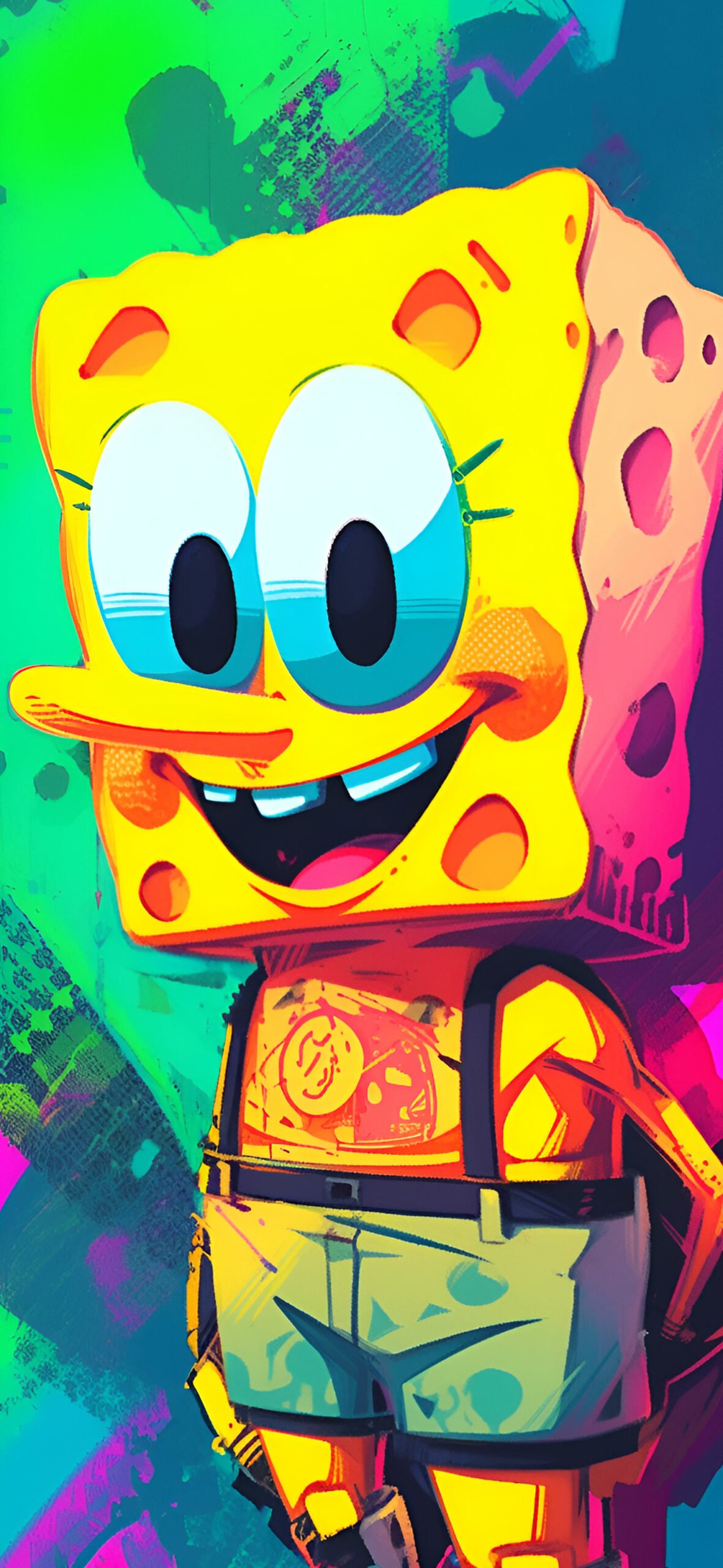The image showcases an animated portrayal of SpongeBob SquarePants, whose iconic square-shaped yellow head resembles a sponge or cheese. His large oval eyes have blue at the bottom with black pupils, and his wide smile reveals three teeth and a visible tongue. SpongeBob in this artwork has a more human-like body with realistic proportions, distinct from his typical cartoonish appearance where his head usually seems larger in comparison. He is clad in black-trimmed jean cut-offs with suspenders over his shoulders and a simple white t-shirt. The background is vibrant and colorful, dominated by green hues on the left, transitioning to blues and some iridescent purples. The right side of the background features more blue, creating a dynamic contrast behind the character. His legs and long nose are also yellow, and his chest is bare with subtle pink and yellow tones.